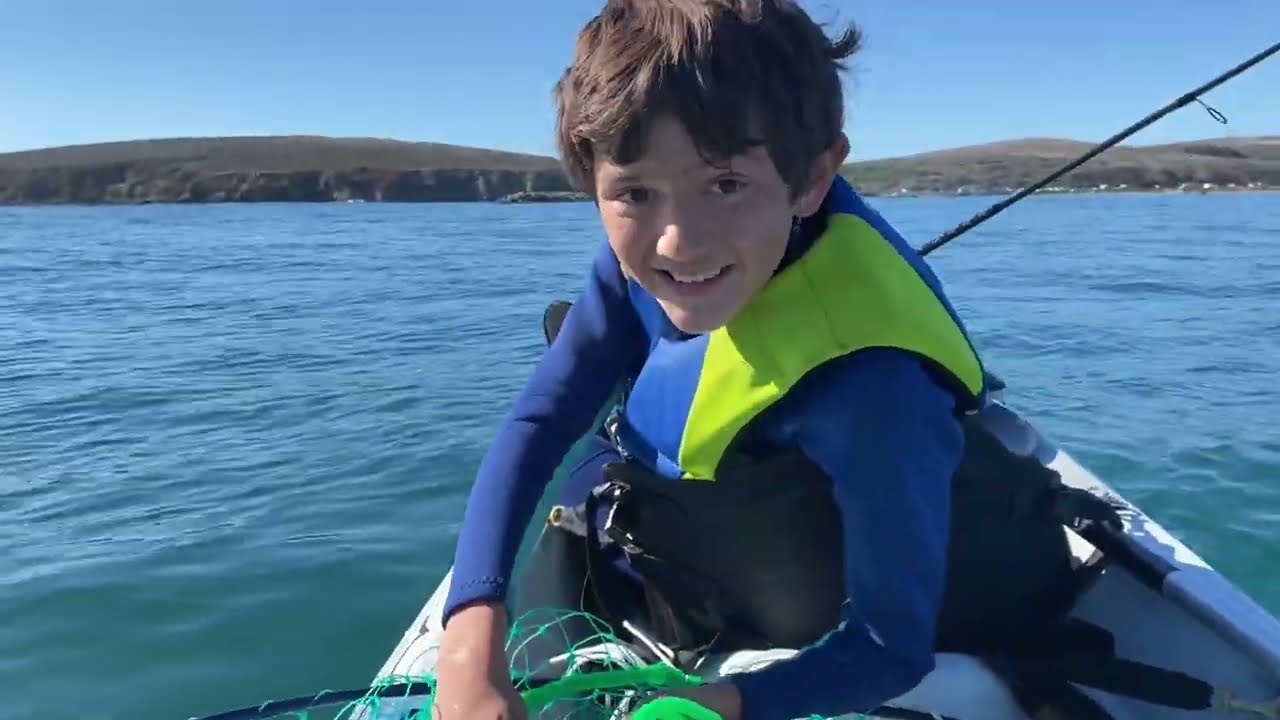In this captivating image, a young boy with brown hair and bangs smiles warmly as he sits in a white canoe or kayak, gliding over a calm blue-green lake. He is dressed in a blue wetsuit and wears a highlighter yellow and blue life preserver for safety. The boy is equipped with a fishing rod extending from the front of the boat, indicative of a leisurely fishing trip. Inside the canoe, a green net can also be spotted. He sits in a black plastic chair, looking back contentedly at the camera. The serene setting features a tranquil expanse of water bordered by majestic hills and rugged rock formations in the distance. The sky above is mostly clear, painted a beautiful shade of blue, contributing to the overall sense of peace and enjoyment captured in this moment.